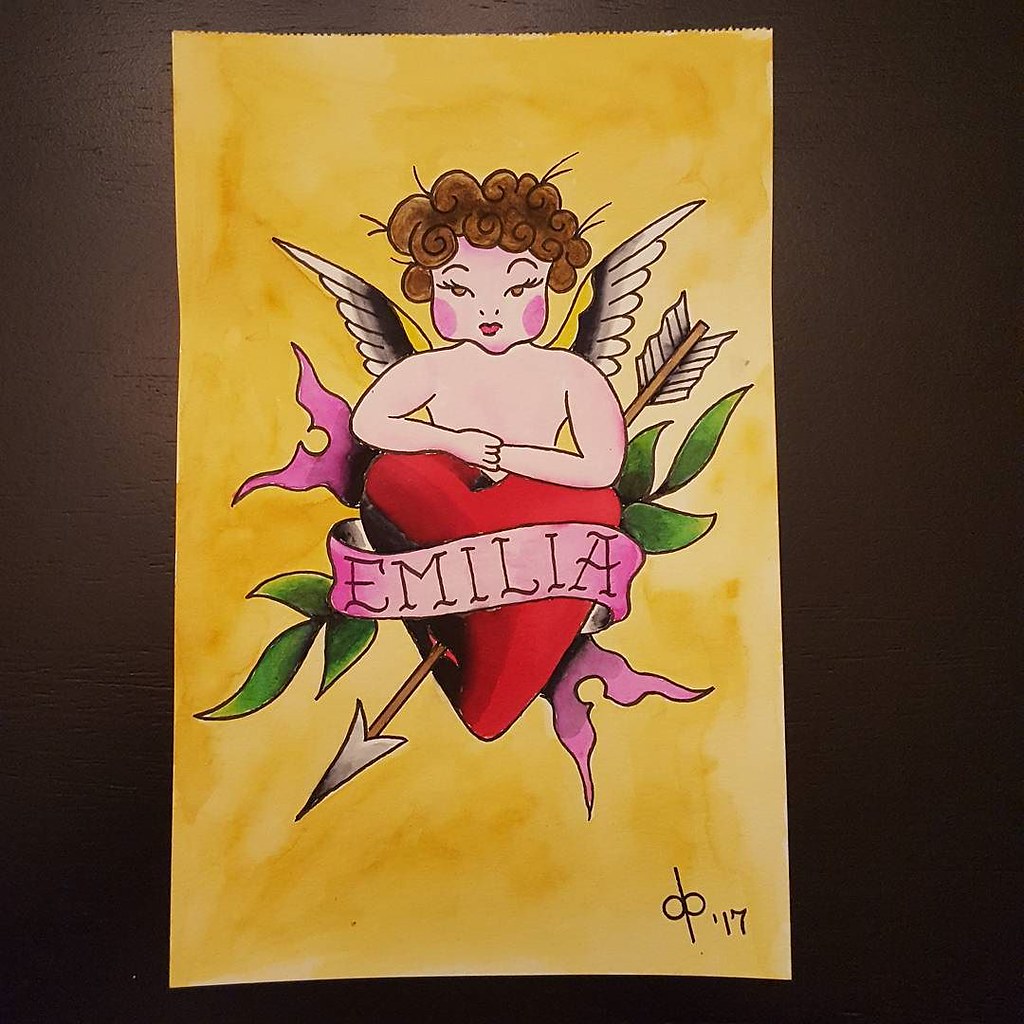This photograph showcases a piece of vintage, old-school tattoo-style artwork. The artwork is resting on a black wooden table, immediately capturing attention with its vibrant elements. The background of the piece is painted a vivid yellow, which contrasts strikingly with the central figure: A solemn angel. The angel, depicted with short curly brown hair and expressive brown eyes, holds a heart pierced by an arrow pointing towards the bottom left corner. Behind the heart, a few artfully detailed leaves add depth and texture to the image. A pink banner, emblazoned with the name "Amelia" in bold black letters, wraps around the heart, its ends visible emerging from behind. The angel's expression is notably unimpressed, with red lips and subtly blushed pink cheeks, contributing to the overall melancholic yet intriguing aura of the artwork.